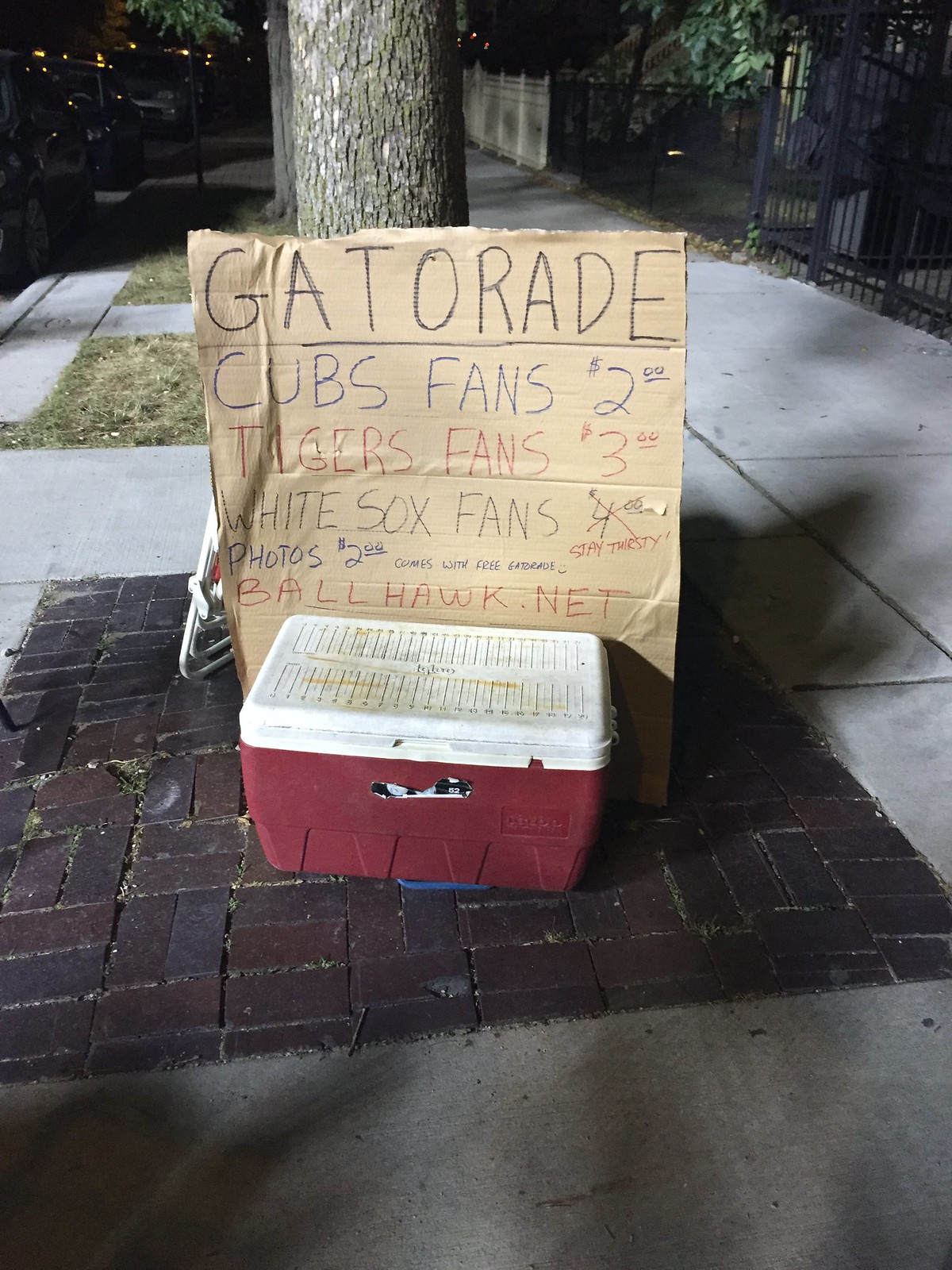The night scene presents a dimly lit street with a tree trunk adorned with mossy patches in the right foreground. A red cooler with a white top sits on a bed of red bricks next to the tree, against a backdrop of thin black metal fences transitioning to white wooden fences in the distance. Beside the cooler, a piece of brown cardboard, propped against the tree, features handwritten text: "Gatorade," followed by "Cubs fans $2," "Tigers fans $3," and "White Sox fans" with "$4" crossed out in red, replaced with "stay thirsty." Further down, the sign reads, "Photos $2, comes with free Gatorade," and "ballhawk.net." A folded chair leans against the tree, while street lights faintly illuminate the scene from the top left corner. This image, likely taken near a baseball game, captures the ambiance of a casual sidewalk setup.